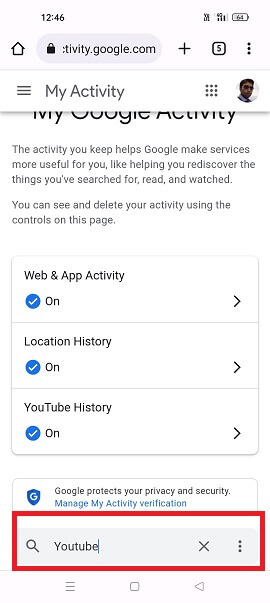A detailed screenshot on a cell phone displays the Google My Activity page. The screenshot shows it’s 12:46 PM and a VoLTE connection with three out of four signal bars. The battery is at 64%. The Google Chrome browser is open to activity.google.com, indicated in the taskbar. The interface includes a menu icon composed of three horizontal lines and the user's profile picture—a mid-30s Indian male wearing sunglasses, looking sideways. 

The visible part of the My Google Activity page contains a paragraph explaining that Google uses stored activity to improve services, helping users rediscover previously searched, read, or watched content. Users can see and delete their activity through the available controls. Below this text, sections include "Web & App Activity," "Location History," and "YouTube History," each marked with a blue checkmark indicating they are turned on. Each section has a rightward arrow suggesting availability of submenus.

Further down, there is a blue shield icon with a "G" indicating Google protects privacy and security, accompanied by the link "Manage My Activity Verification" in light blue. At the bottom of the page, a large red rectangular box overlays a search bar with "YouTube" typed in. The screen's lower section contains navigation icons: three horizontal lines, a Home button, and a sideways triangle for additional menus.